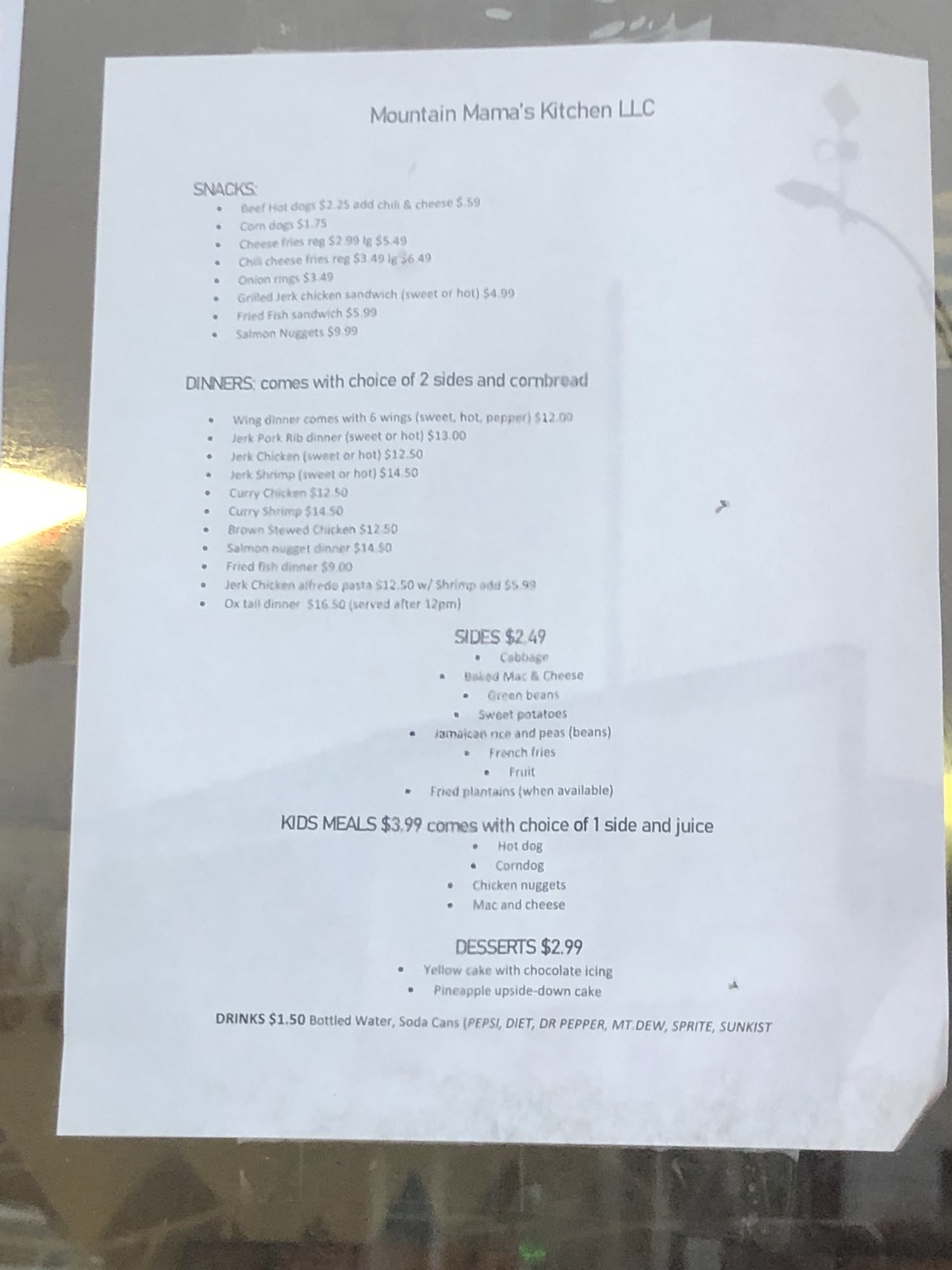This detailed illustration depicts a handwritten menu posted on the window of Mountain Mama's Kitchen LLC, a cozy restaurant with a homey ambiance. The reflection on the glass reveals a glimpse of the street outside, featuring dimly lit streetlights, a nearby building crowned with a flagpole, and the urban buzz surrounding the establishment.

The menu itself is segmented into several sections outlined meticulously: Snacks, Dinners, Sides, Kids Meals, and Desserts. The Snacks section offers about ten tantalizing options, while the Dinners category presents a variety of 10-12 hearty meals, each accompanied by a choice of two sides and cornbread. The Sides section lists approximately eight delicious accompaniments, the Kids Meals feature four thoughtful selections, and there are two enticing items under Desserts.

At the bottom of the menu, there is a clear note stating that all drinks are priced at $1.50. The beverage options include bottled water, soda cans, and a selection of Pepsi products, explicitly noting that no alcoholic beverages are available.

Highlighted dinner options provide a diverse culinary adventure, featuring dishes like Jerk Chicken, Curry Chicken, Curry Shrimp, Brown Stewed Chicken, and a Wing Dinner that includes six wings in your choice of sweet, hot, or pepper flavors, priced at $12. Sides to complement these meals include Cabbage, Mac and Cheese, Green Beans, Sweet Potatoes, and Jamaican Rice and Beans, among others.

Overall, this menu promises a welcoming and flavor-rich experience at Mountain Mama’s Kitchen LLC, inviting patrons to indulge in a variety of comforting and savory dishes.